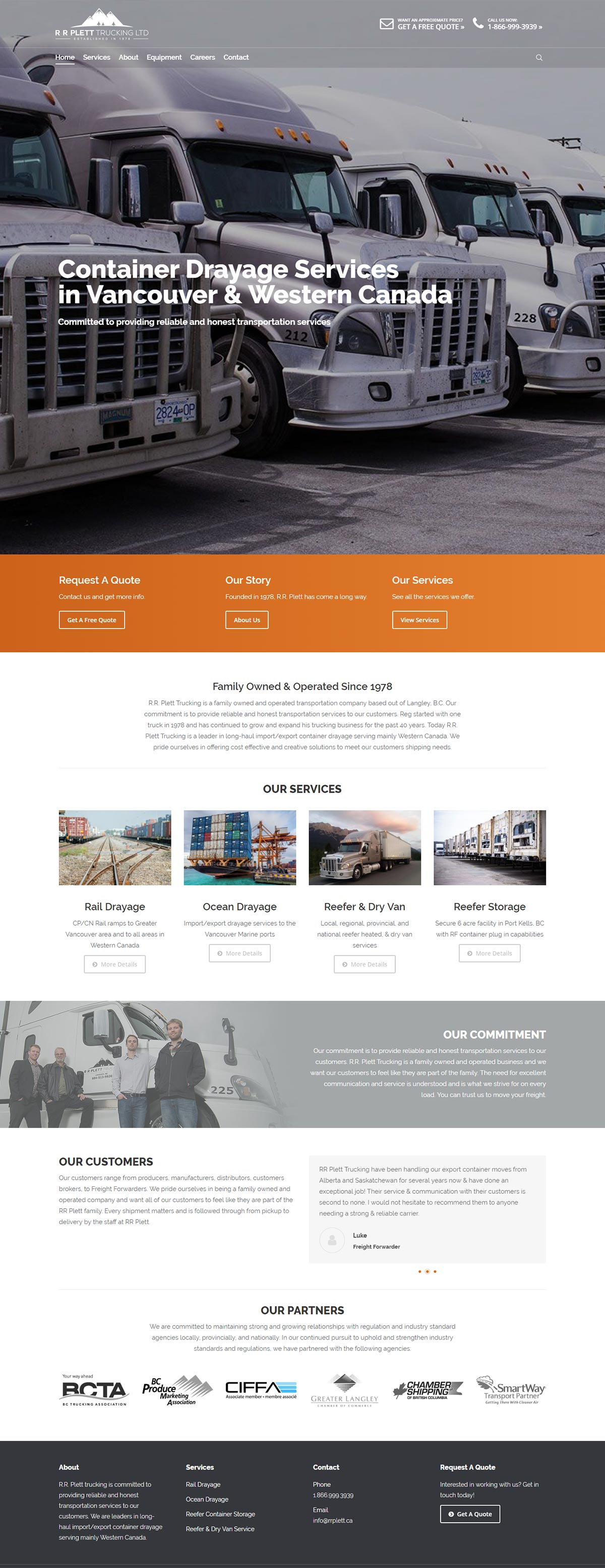In this image, we are looking at a website screenshot. At the top of the image, there is a photograph showcasing a line of truck cabs, including two silver trucks and two white trucks. Prominently displayed in large white text in front of the trucks, the slogan reads "Container Drayage Services in Vancouver and Western Canada. Committed to providing reliable and honest transportation services."

In the upper left corner of the screenshot, there is a logo featuring mountains and trees in white. Below the logo, the company name "Plett Trucking Limited" is displayed. 

Just beneath this visual header, a horizontal navigation bar is visible, filled in a darker gray color. It reads from left to right: "Home," "Services," "About," "Equipment," "Careers," and "Contact."

In the upper right corner of the screenshot, there is a button labeled "Get a free quote," followed by the prompt "Call us now" and the contact number "1-866-999-3939."